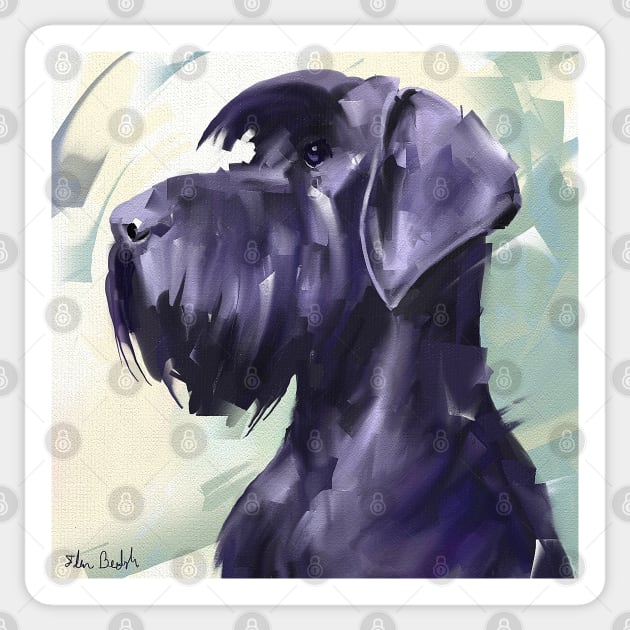This image showcases a hand-brushed, artistic interpretation of a black terrier with long, shaggy fur rendered in broad, abstract strokes. The dog, exuding a calm demeanor, is depicted in a profile view, looking to the left. It has large, droopy ears that hang near its jaw, black eyes, and a blackish-gray nose. A small fringe of hair falls over the front of its face without obscuring it. The background features a gradient of light yellow to light celadon green, framed by a half-inch white border. A cursive signature in black text is located at the bottom left corner, though it is somewhat difficult to read. Across the entire image, numerous watermark emblems, resembling padlocks, are present, indicating it is a stock photo.